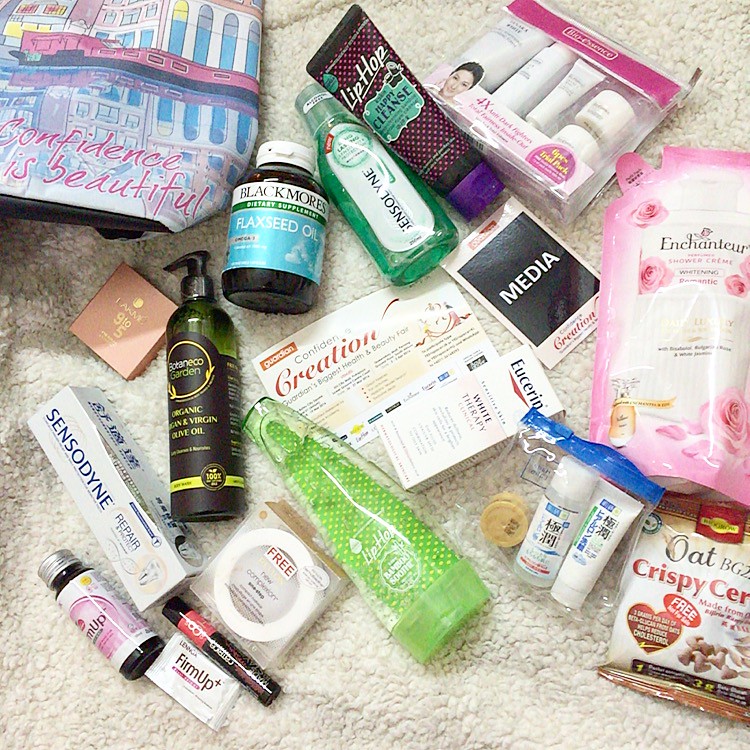The image depicts a chaotic but intriguing assortment of various personal and feminine items sprawled across a white wool cloth. The scene initially gives the impression of a hastily emptied purse, with an array of snacks, toiletries, and cosmetics scattered throughout. 

In the upper left corner of the image, there is a publication titled "Covenants in Beauty," bearing a cover that features an artistic depiction of an old Roman city rendered in pastel colors. 

Adjacent to this magazine or book, there is a bottle of Blackmore's Flaxseed Oil and a small bottle of Sensodyne green mouthwash positioned next to it. Further to the right, a tube labeled "Lip Hop Happy Cleanse," designed with black and pink polka dots and sporting a purple cap, makes an appearance.

Continuing to the right, a prominent pink package containing four or five white bottles, possibly facial cleansers, stands out among other items. The collection includes various hair sprays, lotions, additional toothpaste, lip balm, and soaps, alongside packets of oatmeal and other snack items.

Altogether, the assortment of objects laid out on the wool cloth weaves a detailed narrative of daily essentials and beauty products, hinting at the everyday life and routine of an individual.